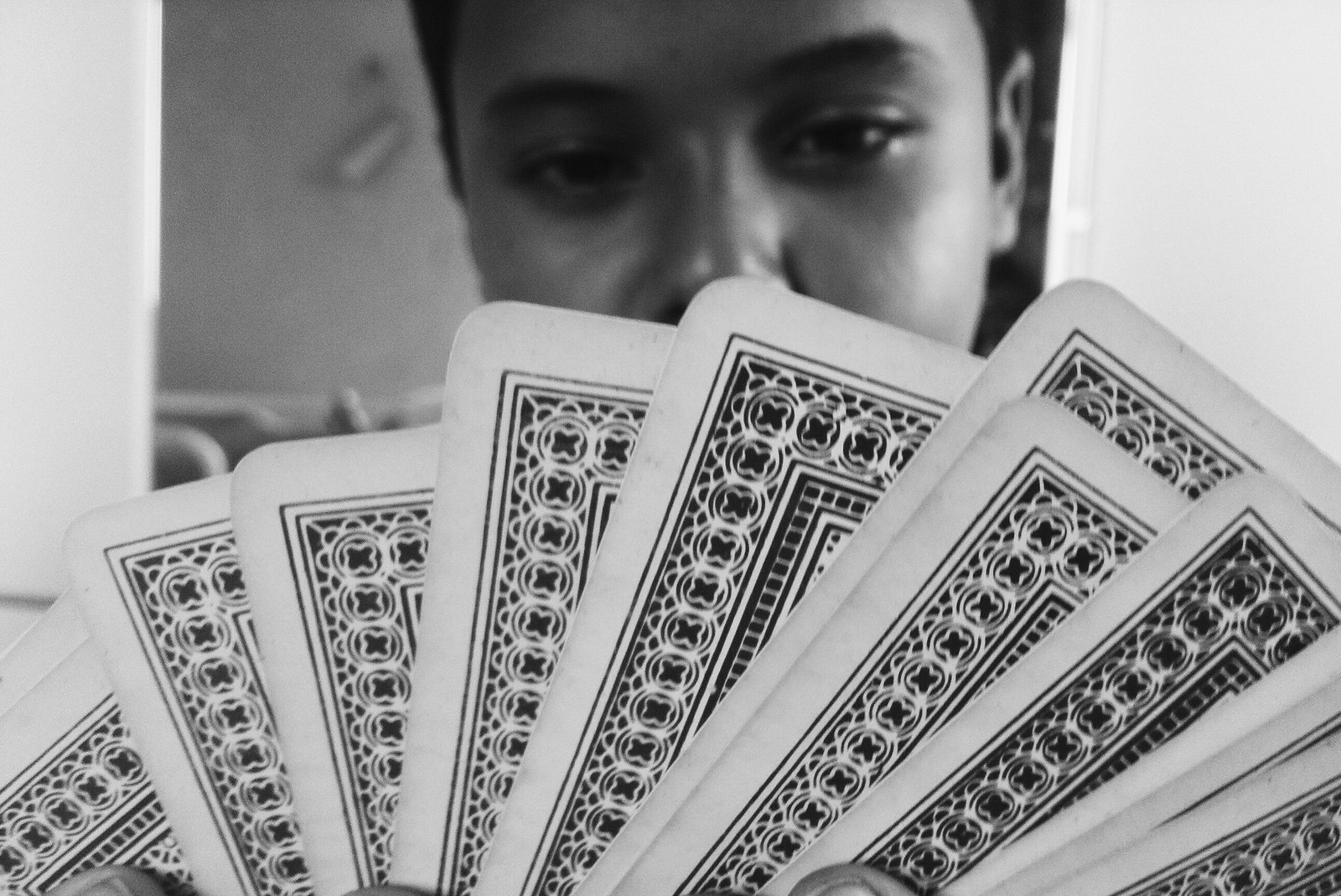In this evocative black and white photograph, an Asian woman holds up a fan of playing cards to the camera, obscuring her mouth. The focus of the image is sharpened on the cards she holds, revealing them as slightly worn with scuff marks, indicating they have been well-used. Only the tips of her fingers, delicately grasping the cards, are visible, contributing to the sense of mystery. The cards are held with a casual disorganization, suggesting an active, ongoing game where cards are frequently exchanged. In the blurred background, a hallway or doorway leads to a darker, indistinct room. The walls are rendered in light gray tones, barely distinguishable due to the out-of-focus nature of the scene. The woman's tan complexion, dark hair, and expressive eyebrows are discernible, despite being out of focus, adding to the atmospheric quality of the photograph.